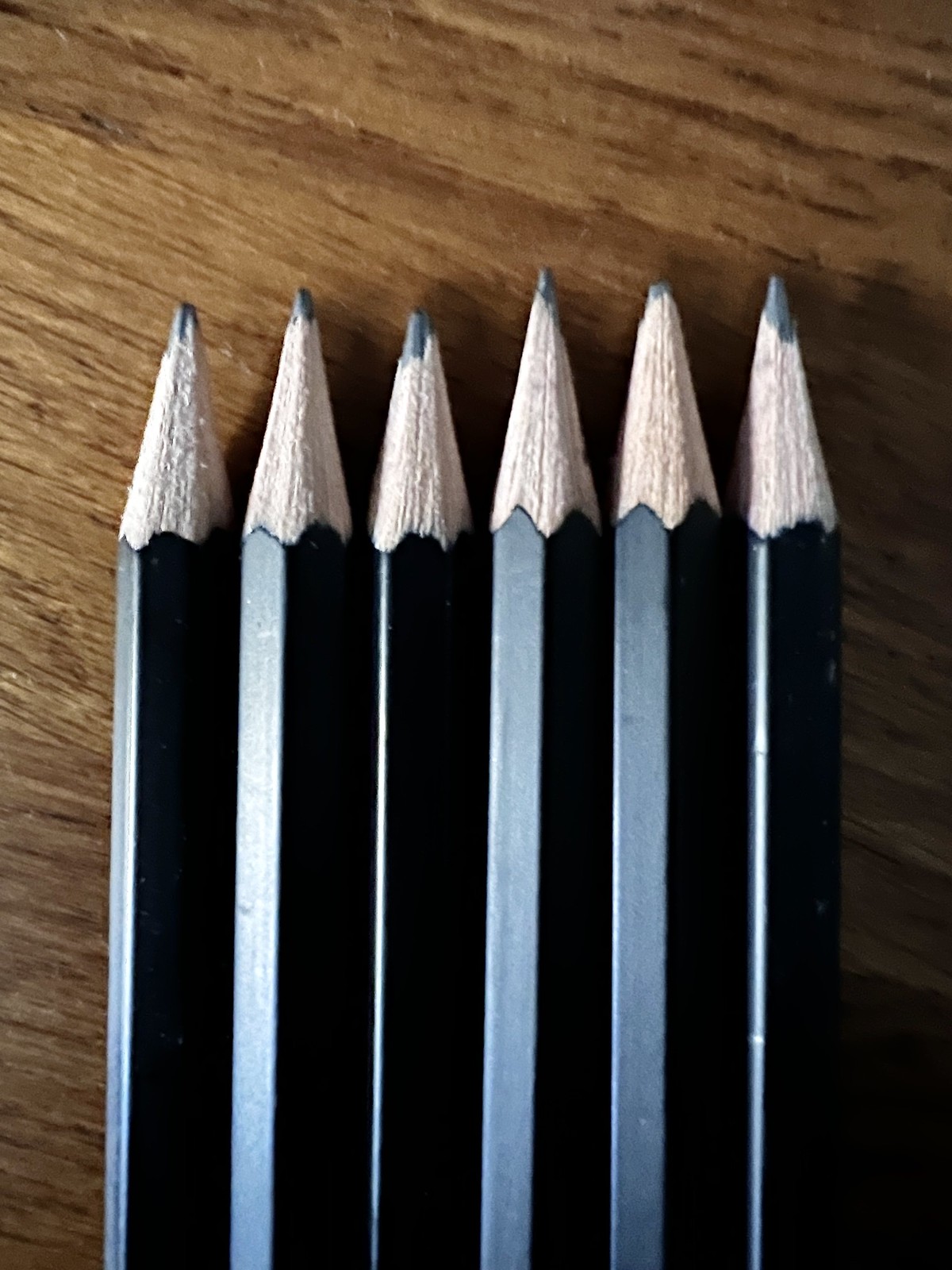This close-up indoor photograph showcases six new, black wooden pencils with graphite tips, meticulously arranged in a vertical row on a natural wooden desk. The pencils are evenly aligned, with their sharpened ends displaying the exposed tan wood and graphite points. Ranging from very sharp to moderately sharp, the graphite tips highlight a slight variation in height—each pencil appears freshly sharpened, with shiny, unmarred, six-sided bodies indicative of their unused condition. The light source, emanating from the left, subtly reflects off the left sides of the pencils, casting a gentler shadow on the right. The image is sharply focused, allowing the viewer to appreciate the fine details of the wood grain in the desk and the pristine surface of each pencil.